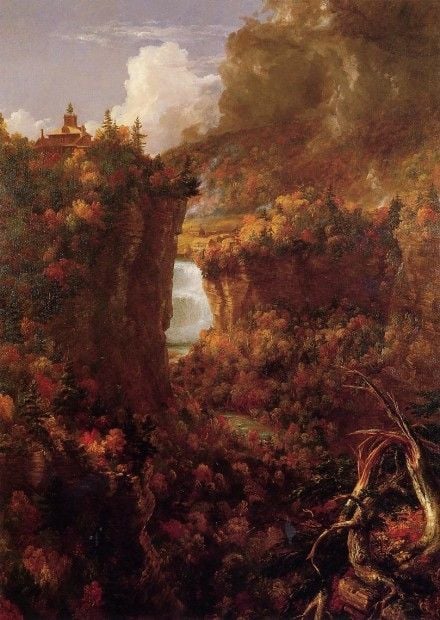This painting depicts a serene mountain valley scene in the fall, characterized by vibrant autumnal hues of orange, yellow, dark green, and dark red. At the very top left of the image, perched on a freestanding hill or cliff, there is a well-maintained house or cottage, though the details of the building are somewhat obscured. The background features a striking blue sky filled with large, billowing white clouds, contrasting with the valley below, which is shrouded in shadows and darker tones. The scene is reminiscent of a setting from a fantasy novel, with rich and dense foliage blanketing the valley. While most of the plant life appears healthy and lush, there is a notable dead tree with a large, broken trunk in the bottom right corner, adding a touch of somberness to the scene. The overall palette of the painting is somewhat muted and dingy, contributing to an atmosphere of calm seclusion.